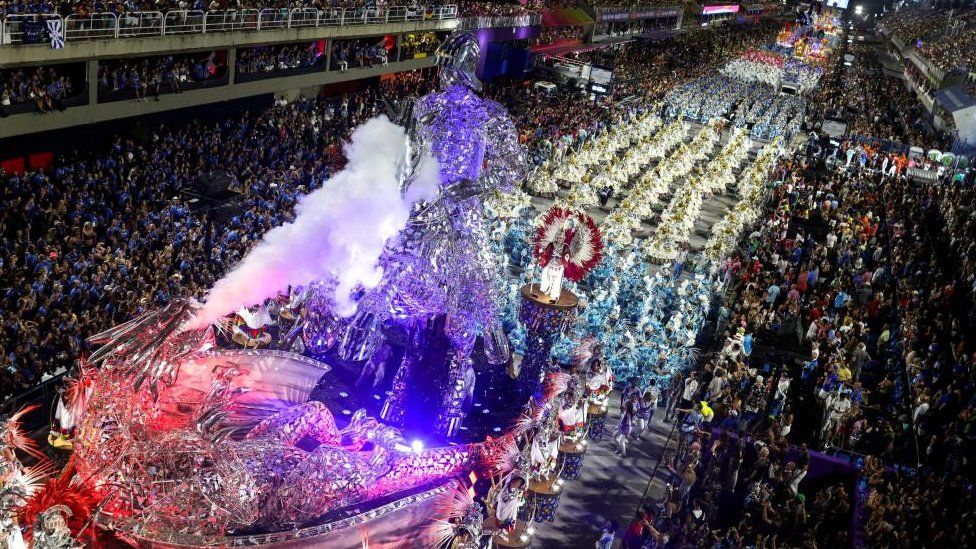This aerial view captures a vividly illuminated parade progressing down a street lined with dense crowds of spectators that extend from the foreground to the background. Positioned at the center of the image is an elaborate float adorned in shades of purple, red, and pink, constructed from materials that create a crystallized effect. The float is set aglow with vibrant lights and emits puffs of white smoke from a pipe, adding to its grandeur. Surrounding the float are numerous participants divided into distinct sections dressed in a variety of colorful costumes, including blue, yellow, white, and red. Onlookers also fill an upper section, which appears to be a balcony, highlighting the extensive public interest in the event. The entire scene is well-lit, providing a dynamic and festive atmosphere.